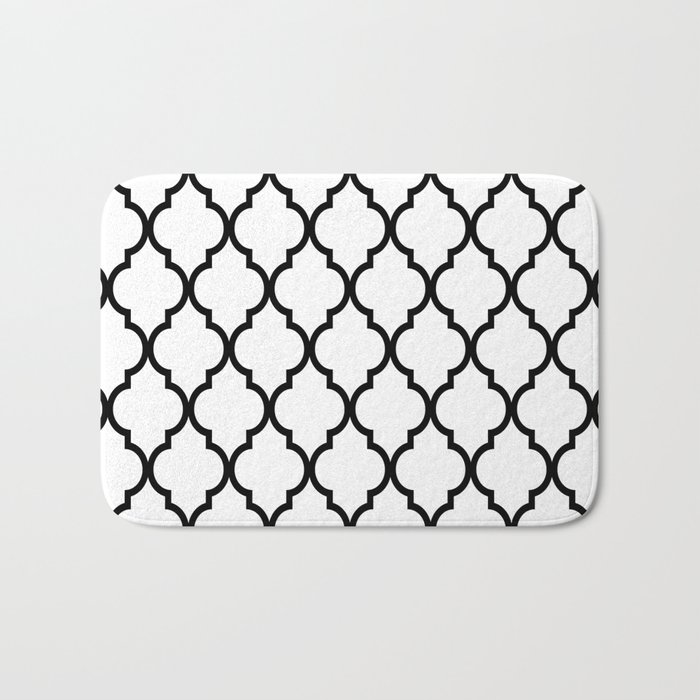The image depicts a small white rectangular rug with rounded edges, possibly used in places such as outside a shower, in front of a sink, or as a cloth placemat. The rug features a soft terry cloth material, hemmed with a loosely stitched edge forming a bead. It has a distinctive black abstract repeating pattern that combines elements reminiscent of spades or keyholes. This intricate black design spans horizontally about five or six times and three times vertically, interlocking seamlessly across the surface of the rug. The rug is laid out on a beige or grayish-beige background, with the rug centered within the frame of the photograph.